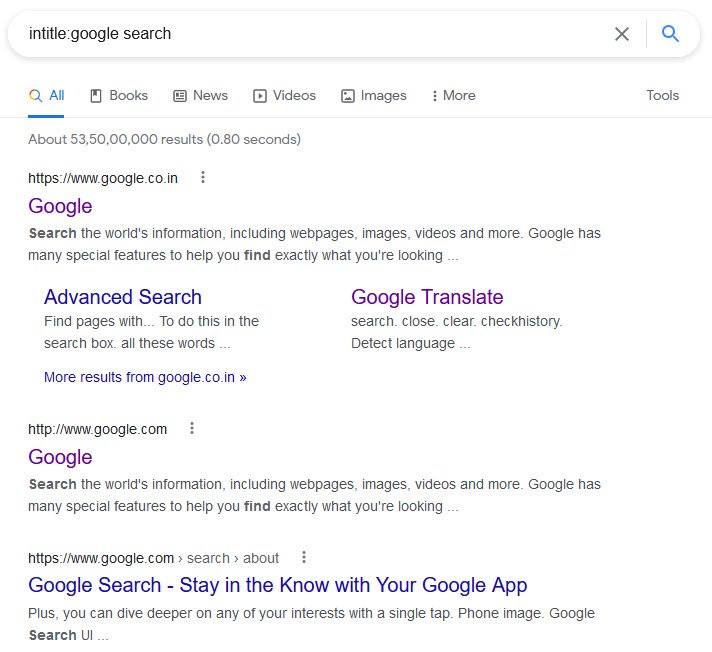The image depicts a basic Google search results page against a white background, featuring the familiar Google logo at the top and the search bar below. The search query entered is "intitle:Google search," utilizing a specific search operator that restricts results to webpages with "Google" or "search" in the title. This filter is designed for more targeted searches. The search results list showcases several links prominently featuring the words "Google" or "search" in their titles, highlighted in blue, with black text descriptions beneath each link. The lack of quotation marks around "Google search" in the query means the results are not limited to pages with the exact phrase "Google search" but include any pages with either "Google" or "search" in their titles.